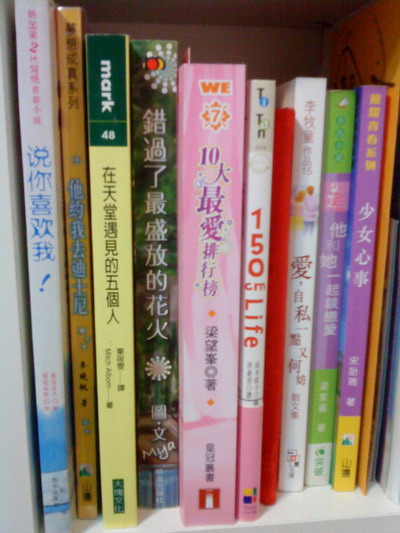This color photograph features a close-up view of a white wooden bookshelf, specifically a single cubicle crowded with an array of ten books. The spines of the books, mostly embellished with Japanese or Chinese characters, are prominently displayed. Each book appears to be unique in design and content, suggesting they are part of different series or topics, possibly Japanese manga or comic books. Among the varied, colorful spines:

- A yellow and green book stands out with the text "Mark 48."
- A pink book, the thickest and most prominent, showcases "W.E. 710."
- A white book titled "150 CM Life" is the only one featuring English text.

Additional books flaunt a palette of hues: one is blue, white, and red; another purely red; a third one combines white, red, and pink tones; there's also a green and purple spine next to a solely yellow book. Although the detailed edges of the bookshelf are barely visible, the neat alignment and vibrant colors of the books present a visually stimulating and organized collection.